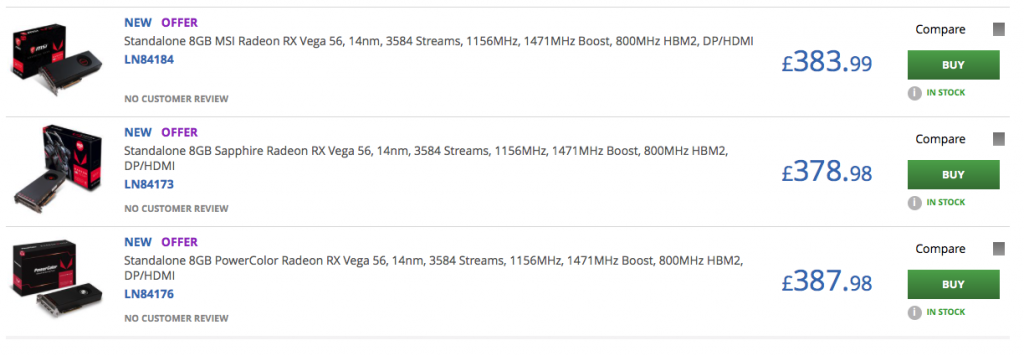This is a detailed caption for an image of a webpage on an e-commerce site selling computer parts:

---

The webpage of an e-commerce website features a clean, white background with text in varying shades of dark gray, blue, and purple. Prices are highlighted in blue. The first item listed at the top of the page is described as "New Offer: Standalone 8TB MSI Radeon RX Vega 56 14NM, 3584 Streams, 1156 MHz Base Clock, 1471 MHz Boost Clock, 800 MHz HBM2 with DP/HDMI." This item—a video card—has a price of €383.99 displayed next to it in blue. To the right of the price, there is a green "BUY" button. 

Items are listed sequentially from top to bottom, all identified as Radeon graphics cards with various specifications and model numbers. The second item is priced at €378.98, and the third item is priced at €387.98. Each price is paired with a green "BUY" button to its right indicating the purchase option.

Below each "BUY" button, in green text, is the indication "in stock," confirming the availability of all items listed on the page.